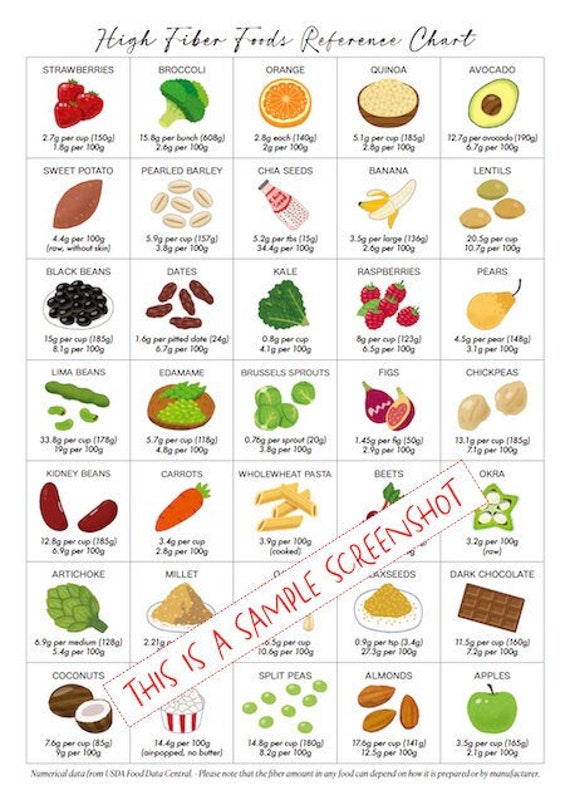The image is a detailed, color screenshot titled "High Fiber Foods Reference Chart" in black letters at the top. It presents a vertical rectangular grid that consists of seven rows and five columns, making a total of 35 sections. Each section contains a food item, starting from strawberries in the top left, followed by broccoli, orange, quinoa, avocado, almond, sweet potato, barley, chia seeds, banana, lentils, black beans, dates, kale, raspberries, pears, blueberries, walnuts, more raspberries, and papaya, among various other fruits and vegetables. Each food item is illustrated with a color image, labeled above in black text, with likely nutritional information written in small text underneath the image, though the latter is too small to read. Diagonally across from the bottom left corner to the upper right is a white banner featuring the text, "This is a Sample Screenshot" in red letters. Beneath the entire grid is small black writing, which is also too small to decipher. The overall layout features a consistent horizontal and vertical alignment of the food items, providing a clear and organized visual reference for high fiber foods.